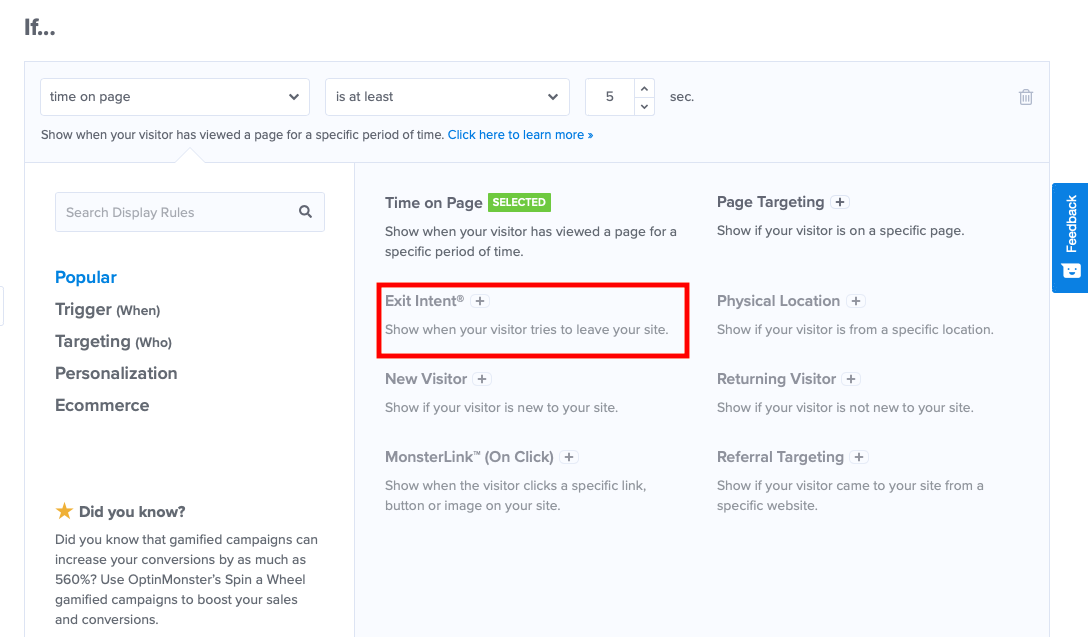This screenshot captures a segment of a website or software interface with a predominantly pale blue background. At the top, in gray text, it displays "If...". Directly below, in a white rectangle, the text reads, "Time on page is at least 5 seconds. Show when your visitor has viewed a page for a specific period of time. Click here to learn more."

The left side features a vertical, white column, which contains several sections. At the top, labeled "Search Display Rule," the sections proceed with labels reading "Popular," "Trigger," "When," "Targeting," "Who," "Personalization," and "E-commerce." Towards the bottom of this column, a star icon accompanies a message stating, "Did you know? Did you know that gamified campaigns can increase your conversions by as much as 560%? Use Opt-in Monster’s spin-a-wheel gamified campaigns to boost your sales and conversions."

To the right of this column, over the pale blue background, the text "Time on page" is highlighted, with the note, "Selected: Show when your visitor has viewed a page for a specific amount of time." Below this, a red rectangle highlights the next option, "Exit Intent Plus: Show when your visitor tries to leave your site." Further down, the options read, "New Visitor: Show if your visitor is new to your site," "Monster Link On Click: Show when the visitor clicks a specific link, button, or image on your site."

In the far-right column, the text includes "Page Targeting: Show if your visitor is on a specific page," "Physical Location: Show if your visitor is from a specific location," "Returning Visitor: Show if your visitor is not new to your site," and "Referral Targeting: Show if your visitor came to your site from a specific web page." A blue rectangle labeled "Feedback" with a chat box icon appears on the extreme right side of the screenshot.